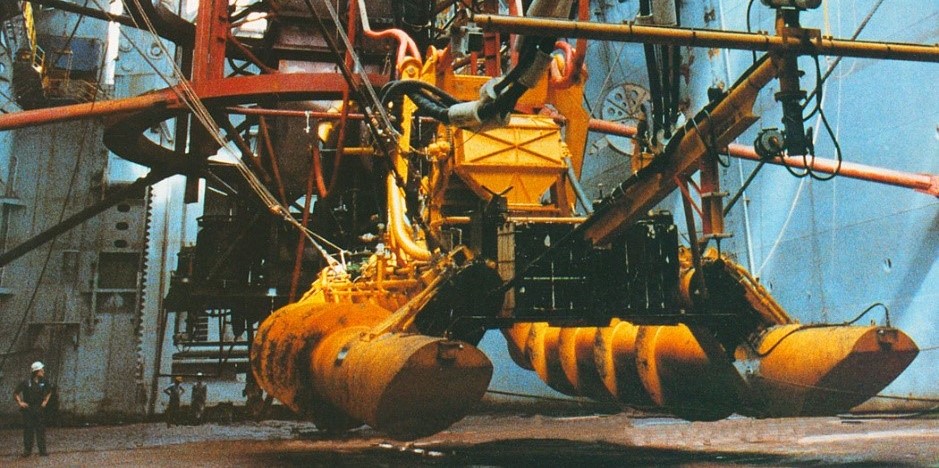The image depicts a yellow submersible machine designed for oil drilling, currently being lowered from a crane on an oil drilling rig. The submersible features two large pontoons, allowing it to float, and its structure narrows from a bulbous rear to a slimmer front. It is encased in steel girding and has a central square area, likely for a control seat. A yellow arm extends from the machine, currently stationary. The scene is set on a large ship with blue sides and an extensive ladder. One man with a white safety helmet stands at the bottom left corner, hands on hips, observing the operation. In the background, additional crew members can be seen, along with the wheelhouse on the left side of the ship.